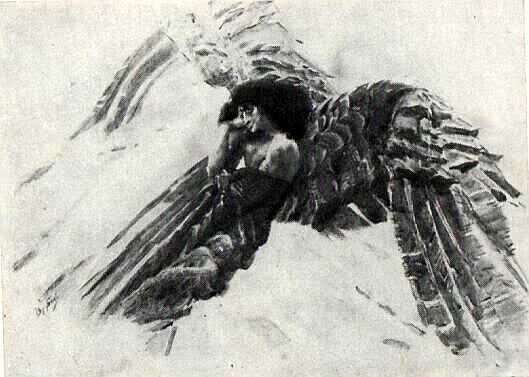This artwork appears to be a detailed, monochromatic charcoal sketch of an angelic figure. The angel is depicted as a man with long, dark, puffy hair, and his face has a bird-like quality. The character's right hand rests thoughtfully on his chin, and he has exposed shoulders and part of his chest visible. He is draped in what appears to be a dark, black fabric or possibly feathers that cover his lower half. He is adorned with large, ornate wings that are predominantly black but show a variance in shading with some sections more densely colored than others, revealing delicate feather details at their ends. The background is primarily a blend of white and gray, with black splotches scattered around, creating an abstract and stark contrast that emphasizes the angelic figure soaring towards the top right corner of the image.